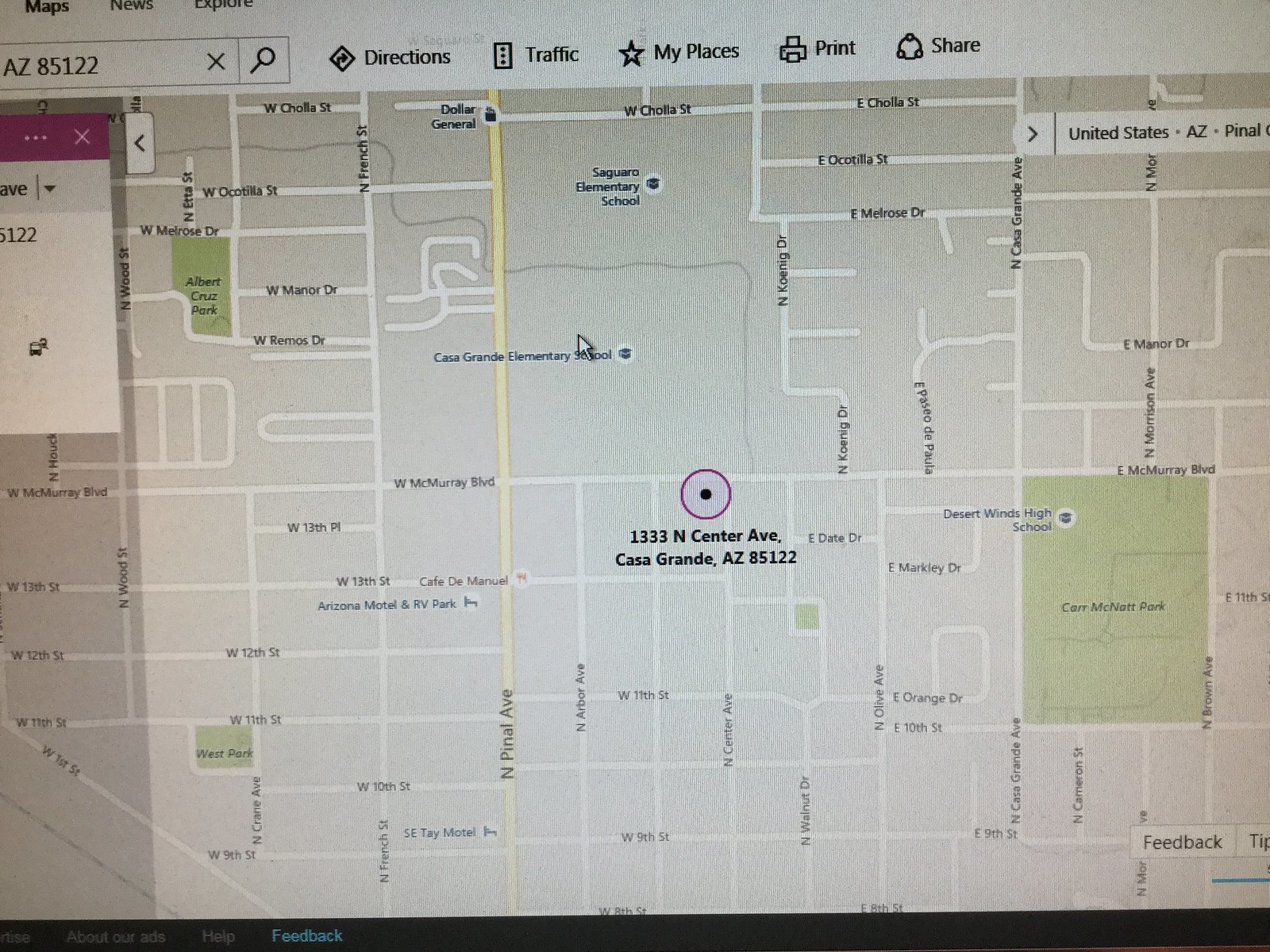This photograph captures a computer monitor displaying a Google Maps window. The map search featured on the screen is for the address "1333 North Center Avenue, Casa Grande, Arizona 85122." The image is not a direct screenshot but rather a photo of the screen taken by someone using a camera or phone. Despite its simplicity, the photo clearly shows detailed mapping and navigation options offered by Google Maps, including the specific location input evident in the search bar at the top of the window. This image illustrates a practical use of digital mapping technology to pinpoint an exact address in Casa Grande, Arizona.